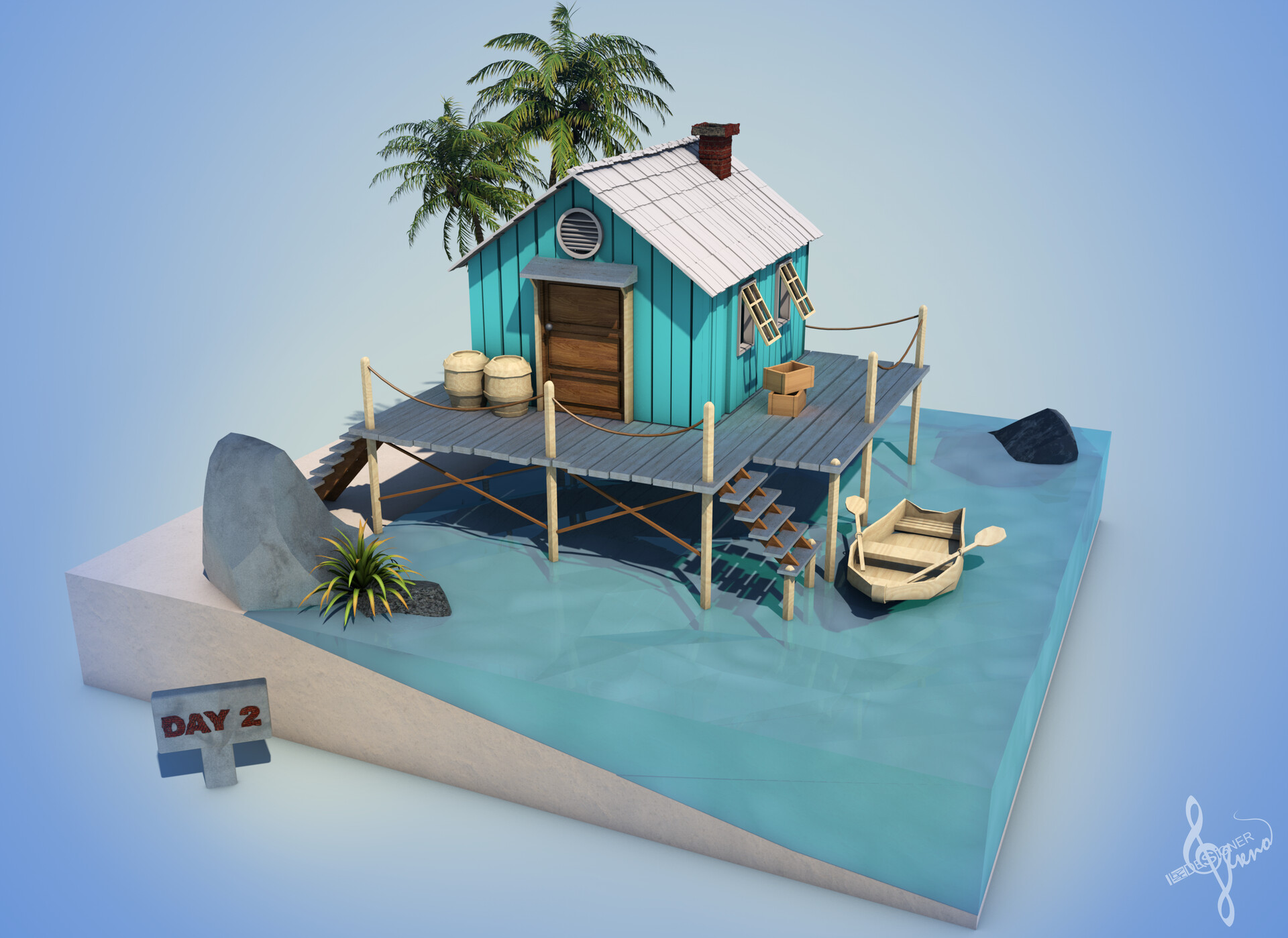The image features a detailed artistic representation of a beach scene set against a light blue background that transitions to white towards the middle. In the bottom left corner, there is a small sign displaying "day two" in red. The centerpiece is a cross-section of sandy land partially submerged in water, containing various elements meticulously arranged. Dominating this section is a quaint turquoise beach hut with a white roof, constructed from vertical slats. The hut boasts open yellow windows, a brown door, and two cream-colored barrels in front. Surrounding it is a gray deck crafted from wooden slats, with steps descending into the water where a small cream-colored paddleboat is moored. Behind the hut, two green palm trees add a tropical flair. Additional details include a rock and an agave plant on the left side, highlighting a blend of natural and man-made elements in a miniaturized beach setting.